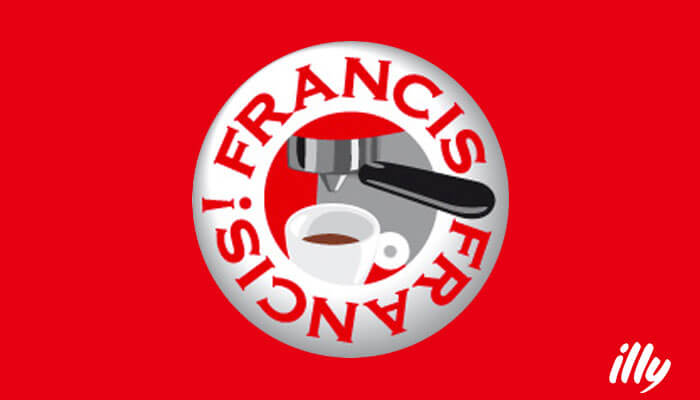The image depicts a predominantly red logo with a central white circle featuring an illustration of an espresso machine spout and a white coffee cup with a bit of coffee at the bottom. Surrounding the illustration, the words "Francis Francis!" encircle the border of the circle. The espresso machine illustration highlights a black handle and a silver spout, emphasizing the coffee being poured. In the bottom right corner of the image, the brand name "illy" is written in a calligraphy-style lowercase font. The overall design is clean and conveys a strong brand identity.